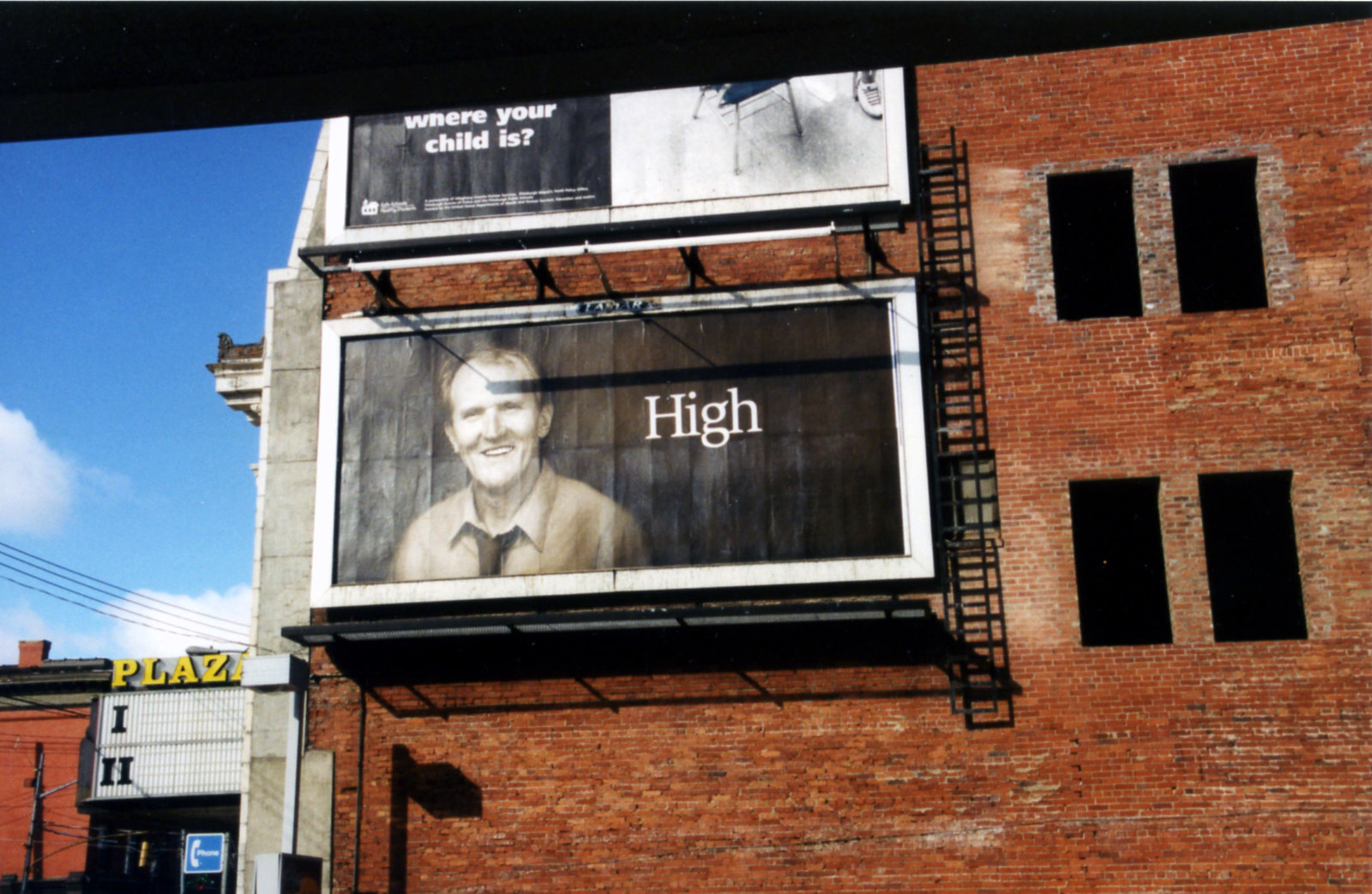The image captures the side of an abandoned, industrial-looking red brick building. The building, which is two stories high with black-covered window openings, features two rectangular billboard advertisements mounted one above the other. 

The lower billboard presents a middle-aged man in a brown shirt and black tie, smiling against a black background, with the large white letters "HI" to his right. The upper billboard, partially visible, has a similar black-and-white color scheme and reads "WHERE YOUR CHILD IS?" in white letters against a black background, with what appears to be a chair next to the text. 

Both billboards are fitted with railings and a ladder on the right-hand side, accompanied by a platform for maintenance access. The structure suggests they are regularly changed, likely by advertising personnel. 

Adjacent to this building, to the left, there's a glimpse of a blue sky with white clouds, and part of another structure, identified as "Plaza" by its large yellow letters. Below "Plaza" are Roman numerals I and II, hinting at sections or floors, alongside a sign depicting a telephone, with a blue background and white lettering indicating the presence of a phone service nearby.